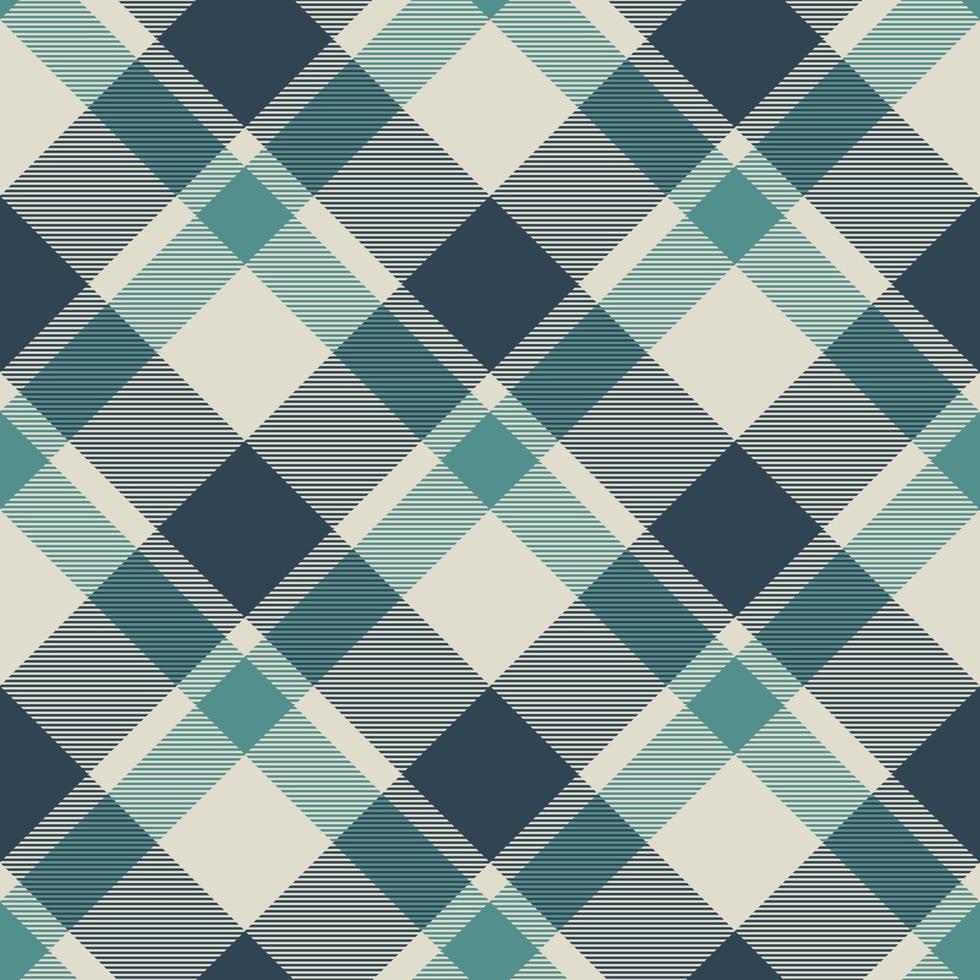The image showcases a fabric adorned with a detailed and seamless plaid pattern, which could be used in clothing design. The pattern predominantly features a series of intersecting lines in various shades of green, teal, and dark blue. Dark green, lighter green, and a creamy white color form the checkered foundation of the design. Thin horizontal and diagonal lines in green and dark blue intersect, creating distinct blocks of color. Where the green lines cross, they form thick green squares, and the intersection of the blue lines results in dark blue squares. Additionally, when teal lines intersect, they produce solid teal squares, and where blue and teal lines overlap, they create dark blue and teal rectangle shapes. The design is simple yet intricate, with repeating elements that would align seamlessly if tiled.